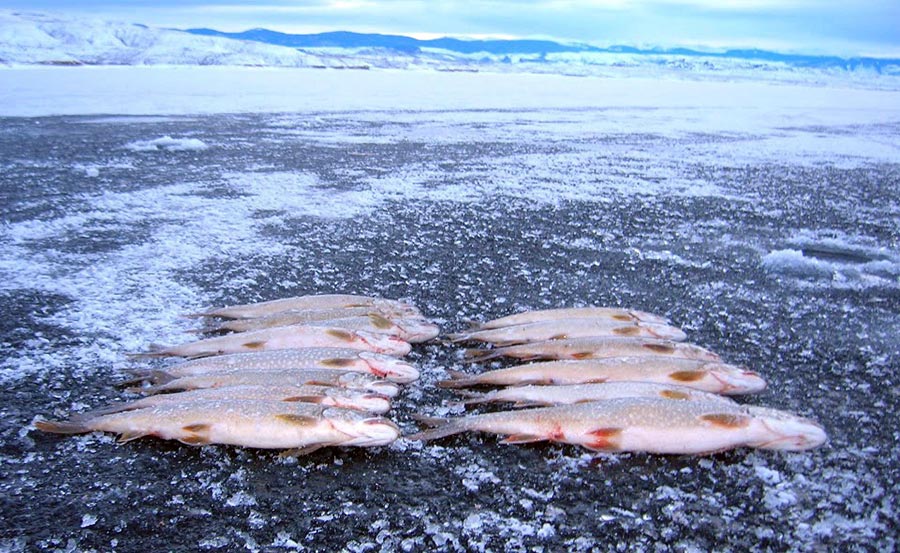This outdoor photograph captures a cold, snowy wilderness scene with distant mountains under a blue, cloud-strewn sky. In the foreground, lying on a black, rocky surface speckled with snow, are twelve pale, light pink fish arranged in two meticulous rows. Each row contains six fish, all uniformly positioned with their red-tinged heads pointing to the right and their tails to the left. The fish, varying in shades from gray to white with red spots, are set against the stark, gray-black ground, enhancing their distinct features. The background features a snowy expanse, possibly a frozen or snow-covered body of water, beneath the majestic, darker snow-capped hills and mountains that frame the scene. The overall composition of the photograph highlights the serene yet harsh beauty of this cold environment and the unusual alignment of the fish on the icy, rocky shore.